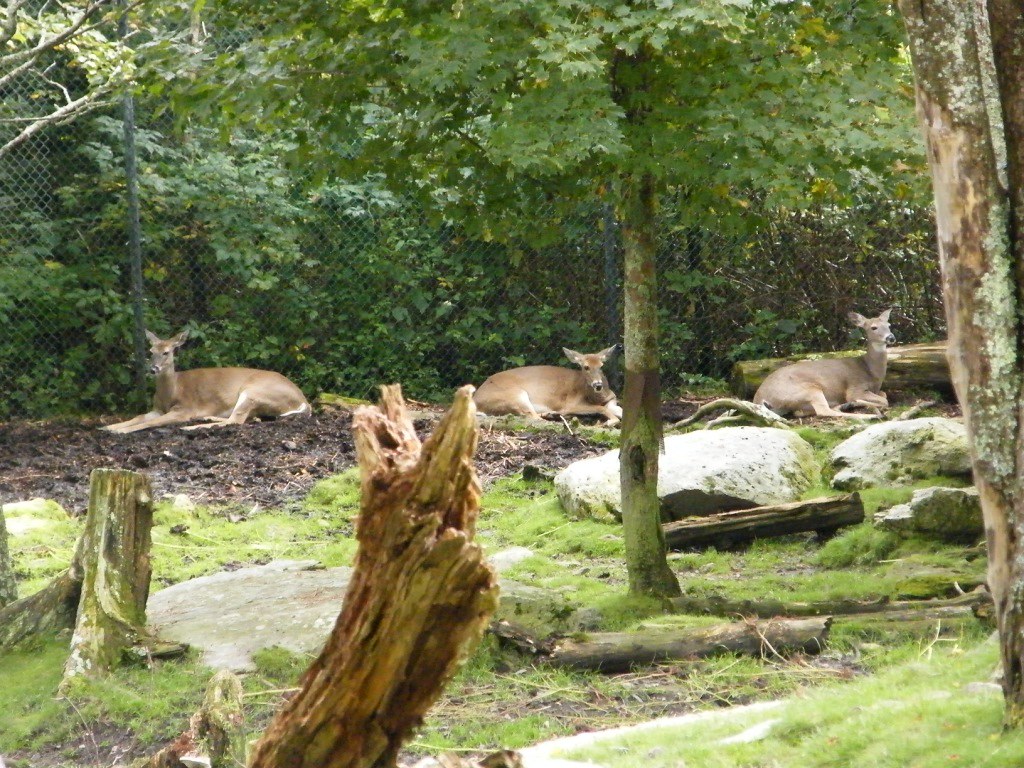In this square-shaped photograph taken in an outdoor setting, three deer—one on the left, one in the middle, and one on the right—are lounging on a heavily soiled grassy area. The background is composed of a green chain-link fence, behind which a dense array of leafy trees can be seen. The deer are surrounded by varied elements of the natural landscape: tree trunks, some broken or cut-off, lie scattered among patches of grass and dirt. On the right-hand side of the image, there is a tree trunk with some greenery around it, and similarly, on the left center, another broken tree trunk is visible. The foreground displays additional vegetation, including a full tree with leaves and some wood and rocks strewn about. The scene is well-lit with natural light, highlighting the tranquil setting despite the overcast appearance.